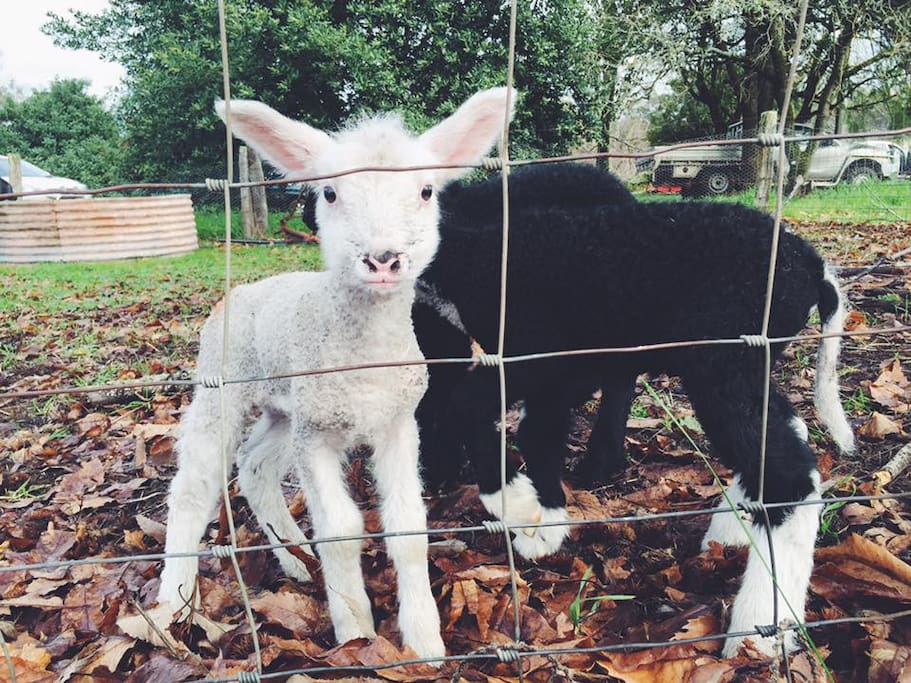The photograph captures a tranquil outdoor scene with three baby goats standing behind a barbed wire fence. The foreground is strewn with brown leaves and patches of green grass peeking through. Among the goats, the one on the left is a white baby goat with pink inner ears, a pink nose, and dark eyes, facing directly towards the camera. Next to it is a slightly larger black goat with distinct white feet and a white tail, turned sideways. The third goat, also black, has its head hidden, adding to the curiosity. In the background, several trees with dense foliage frame the scene, and a silver older-model pickup truck is visible in the upper right corner. Additional elements include a wooden post, a shed, a metal watering bowl for the goats, and a section of metal trim on the fence, enriching the rustic ambiance of the image.